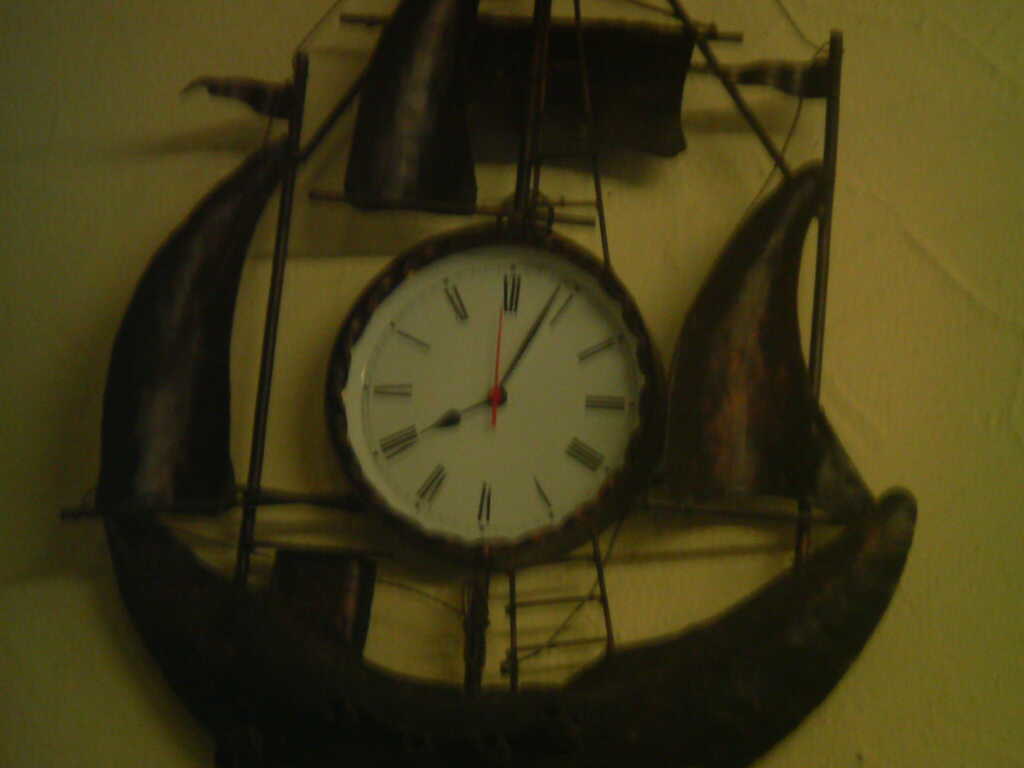This image is a blurred photograph of a white clock hanging on a yellow wall. The clock, designed to resemble an old vintage sailboat, has a round face adorned with Roman numerals. The frame of the clock features a rusted brown, dark bronze metallic material, giving it an aged, weathered appearance. The lower part of the frame is crescent-shaped, imitating the hull of a boat, while the sides and top are decorated with sail-like shapes and flagpoles, enhancing its nautical theme. The clock's hands are black, with a teardrop-shaped hour hand and a straight minute hand, both complemented by a red second hand ticking around the face. The time displayed is approximately 8:04, and despite the dim lighting conditions, the clock and its elaborate boat-like frame are clearly visible in the photograph.